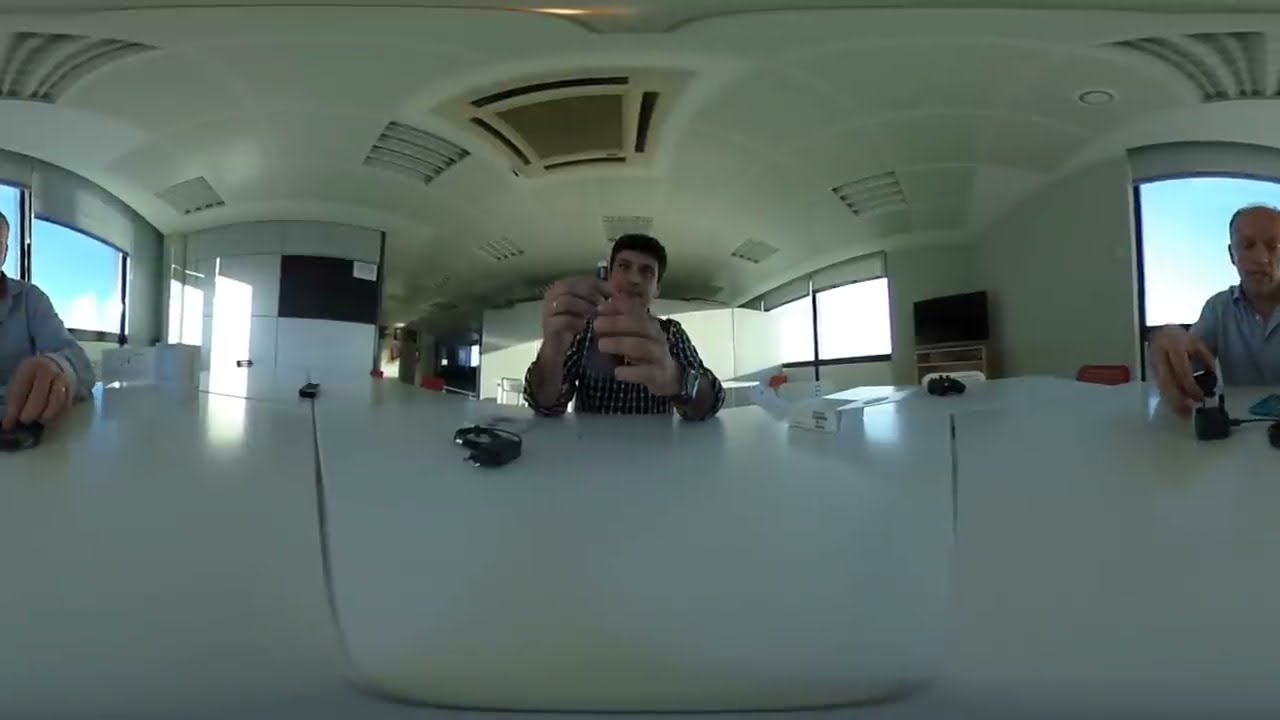In this fisheye lens photograph, the central figure is a Caucasian man with short dark brown hair, wearing a plaid shirt that is a mix of brown, dark green, and possibly some other colors. He sits behind a pristine white modular desk in an office setting. The man appears to be holding a small object—likely a USB plug or possibly a silver nail or flash drive—in his slightly chunky, outstretched hands. The panoramic effect of the image causes the illusion of a second person on both the left and right, who actually seem to be reflections or distortions of the same older, balding Caucasian man, dressed similarly in casual dress shirts. Behind the central figure, the office features a wall of windows showcasing a clear blue sky, indicating it is daytime. The sparse interior is marked by white walls and ceilings fitted with several air vents. A mounted black TV is visible on a white wall to the left, while another TV sits on a small shelf to the right. The surroundings have a somewhat Art Deco appearance with an overall minimalist design. The office is bright and appears to have ample natural light filtering in through the windows.